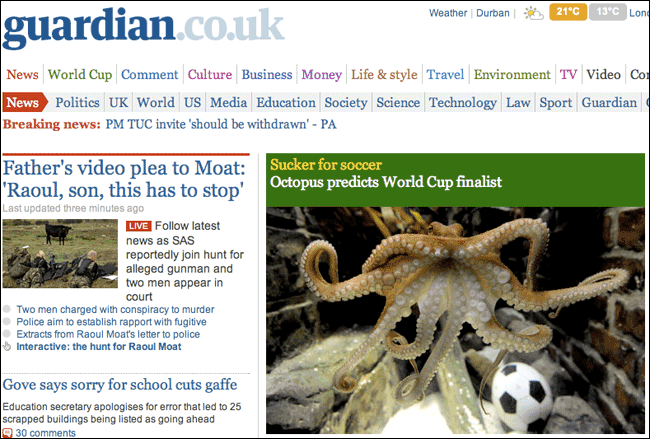This is a horizontally oriented image that appears to be a screenshot of an online publication, accessible via an app, website, or smart device. It has a thin black border encompassing the entire image. At the top of the screen, the website’s address "guardian.co.uk" is prominently displayed, with "The Guardian" in deep blue, bold text, and "co.uk" in a lighter, regular font. In the upper right corner, the current weather in Durban is shown with a partly sunny icon. The temperature options are displayed as 21°C in orange and 13°C in gray.

Below the header, a navigational menu lists various sections: News, World Cup, Comment, Culture, Business, Money, Life and Style, Travel, Entertainment, TV, and Video, although the last word is partially cut off. Clicking on "News" would reveal subcategories like Politics, UK, World, US, Media, Education, Society, Science, Technology, Law, Sport, and Guardian.

The main section of the screen features breaking news with the headline: "PMTUC invite should be withdrawn - PA." Below that, there is an article titled "Father's video plea to Moat: Raul's son, this has to stop," providing details about the plea. Another headline reads, "Government says sorry for school cuts gaffe," with further commentary on the issue.

Central in the image is a photograph of an octopus with a soccer ball, captioned "Sucker for Soccer: Octopus predicts World Cup finalist." This whimsical image appears to accompany a story on the octopus making predictions related to the World Cup.